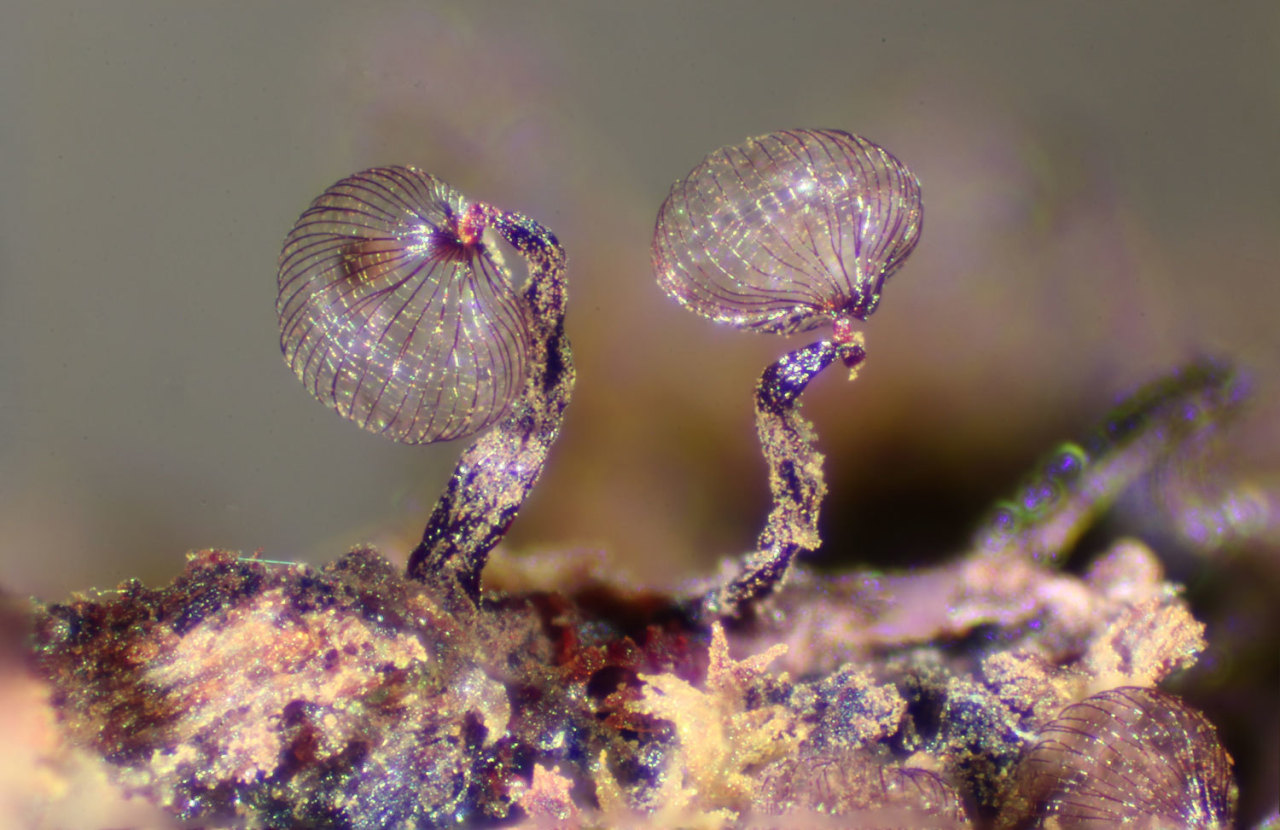The image portrays a detailed close-up of a mysterious specimen, possibly a natural element like a flower or mushroom, set against a blurred, earthy-toned background. The background mutes into gray, brown hues, leaving the focus entirely on the intriguing subject in the foreground. Emerging from an earthy, muddy surface that appears dark brown and black with hints of yellow and tan, two stems rise up. These stems culminate in transparent, jellyfish-like domes, adorned with intricate, thin veins. The domes shimmer with a sparkly, almost glittery appearance, evoking a sense of delicate beauty. The main specimen, seemingly clear or gold-tinted, casts an enchanting glow, with its central positioning complemented by smaller, similar formations branching off to the sides, adding to its elegant and mesmerizing allure.